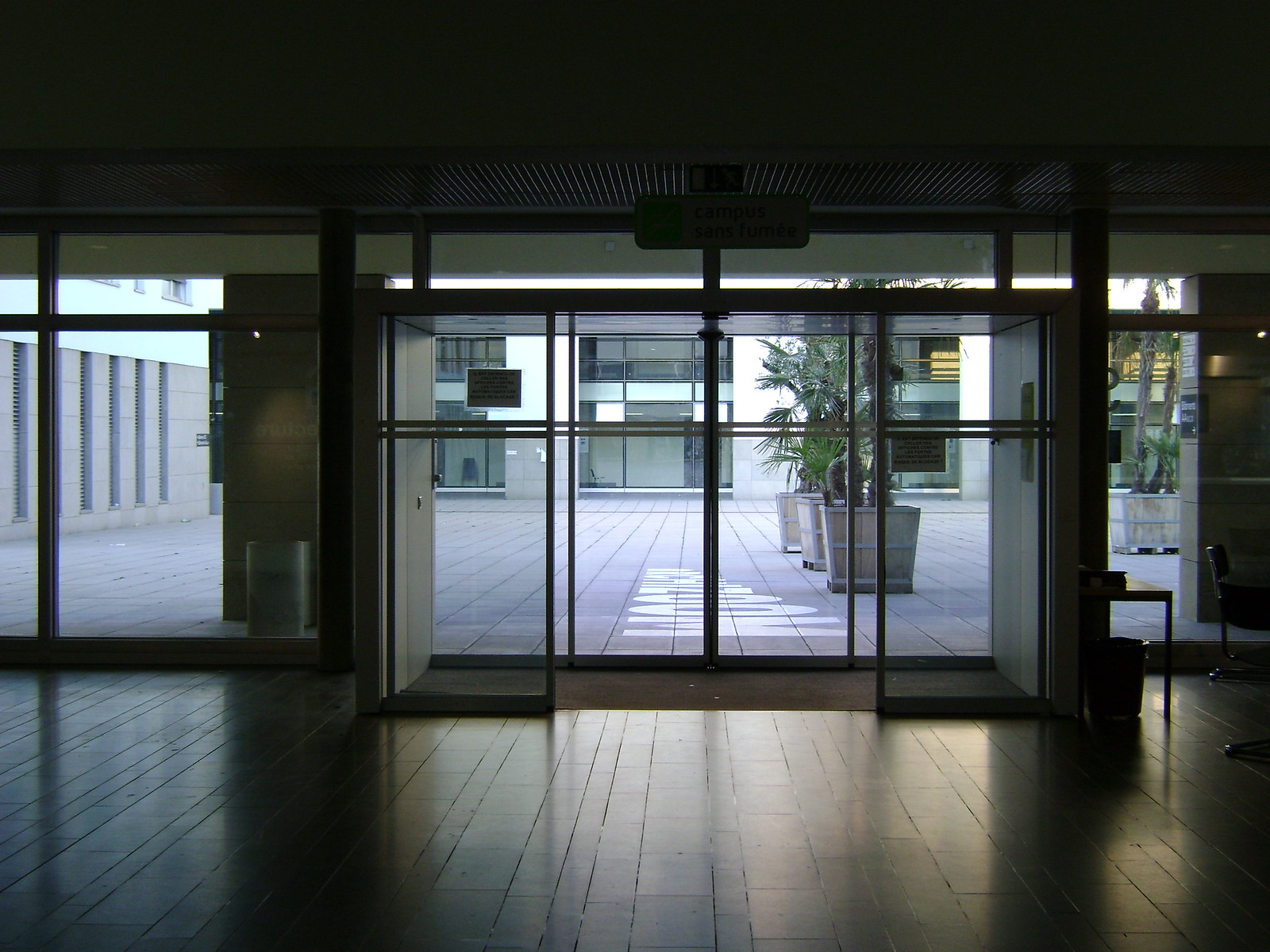The image captures an interior view of a modern and possibly commercial office building, characterized by an expanse of glass walls and glass doors that provide an unobstructed view into an adjacent courtyard. The lower third of the image showcases an indoor area with a gray floor, dimly lit, likely due to the absence of interior lighting. This dark ambiance is contrasted by patches of natural light streaming in through the glass surfaces, creating shadows and reflections on the floor. The middle section prominently features large glass doors, possibly automatic and equipped with multiple panes separated by thin metal bars, leading out to the courtyard. The courtyard itself is minimalist, containing tan plant holders with green plants and trees, and bordered by windows from an opposite building wing in the distance. Signage, perhaps indicating operational hours, can be seen affixed to some of these windows. The top portion of the image is dominated by a black ceiling, further emphasizing the dark indoor setting. This overall scene exudes an air of modernity and professionalism, likely representing a contemporary office or commercial space.